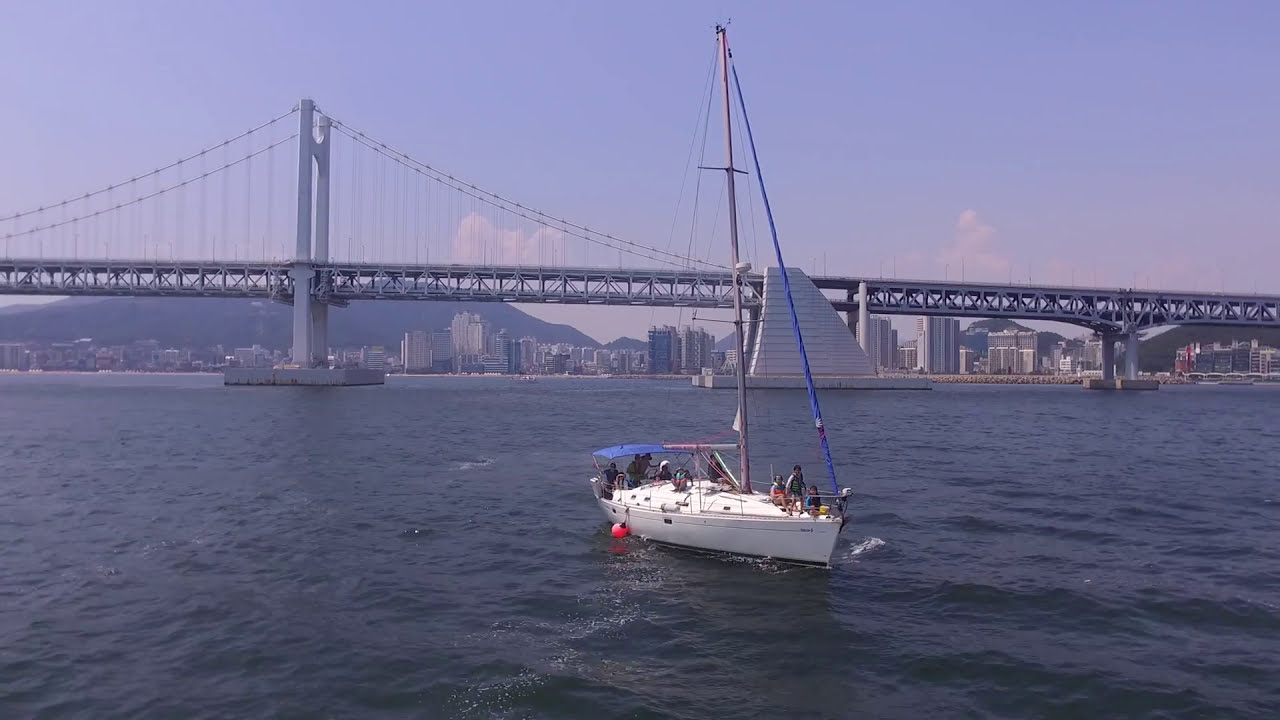In this vibrant outdoor photograph, a white sailboat with its sail down and a blue awning at the back gracefully drifts on dark, wavy water. The boat, populated by around eight or nine people, is adorned with a red buoy on its left side. The clear, sunny day boasts a blue sky accentuated by a few fluffy, low-flying clouds. The backdrop is dominated by a grand suspension bridge, almost certainly the Golden Gate Bridge, with its distinctive cables stretching up into the sky. Beyond the bridge, the skyline of a bustling city features a variety of high-rise buildings of different shapes and sizes. Further in the distance, a rolling hill adds to the picturesque scenery, completing the captivating view.